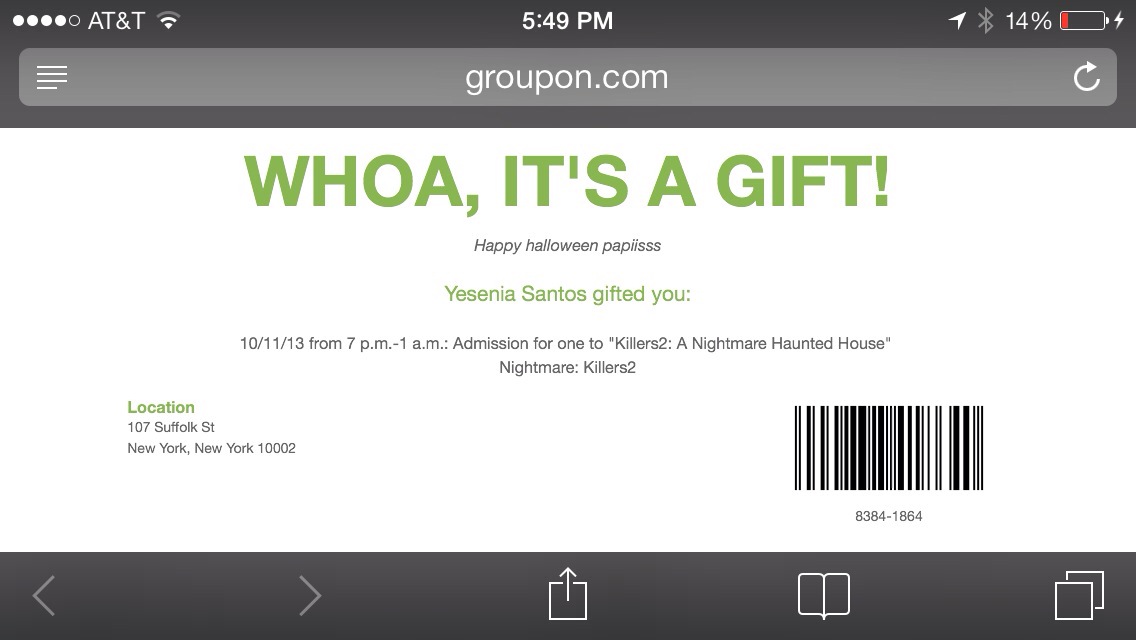A screenshot taken from an iPhone displays a Groupon coupon or gift card on the phone's screen. At the top left, the AT&T carrier is shown with a partially filled signal strength indicator. The time is 5:49 PM, and on the top right, the phone's battery is at 14% and charging, indicated by a red battery icon with a lightning bolt. The webpage is from Groupon.com, as shown at the top. Below that, in bold green letters, it says, "Whoa, it's a gift!" followed by "Happy Halloween, PAPIISS" in small black letters. Further down, in green text, it states, "Yesenia Santos gifted you" and details an event: "10-11-13 from 7 PM to 1 AM, admission for one to 'Kill us Two,' a nightmare haunted house," at the location, "107 Suffolk Street, New York, New York, 10002." At the bottom, there is a barcode for redemption labeled with the number "8384-1864." The main colors on the screen are gray, white, and green, with navigation symbols at the bottom.